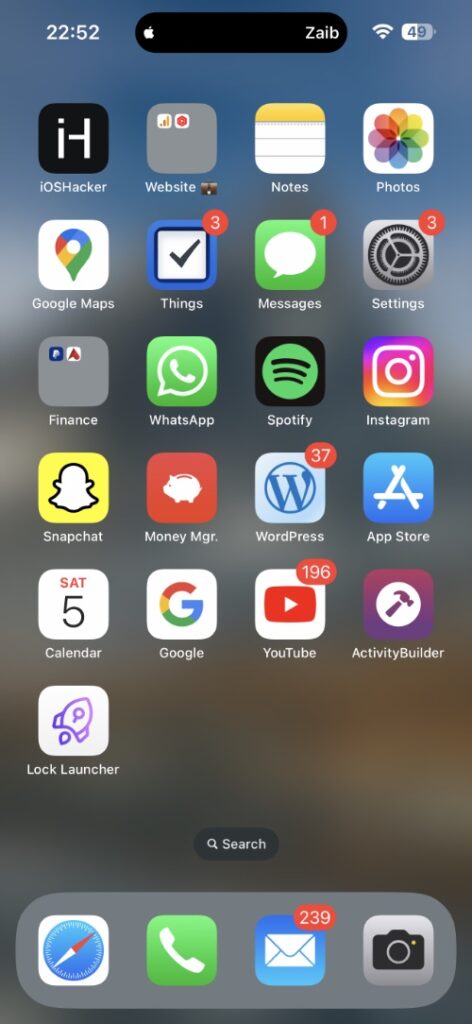The image captures a smartphone screen displaying the time "22:52" at the top, alongside an Apple logo and the label "Zabe." The status bar also features a Wi-Fi indicator and battery percentage. The screen showcases an array of app icons, each distinctly identifiable. 

- **Top Row of Apps**: 
  - **iOS Hacker** app
  - A folder labeled **Website**
  - **Notes** app
  - **Photos** app
  - **Google Maps** app, identified by its colorful pin icon
  - **Things** app, marked with a check mark and the number "3" indicating notifications.

- **Middle Row of Apps**:
  - **Messages** app, showing one new notification
  - **Settings** app, with three notifications
  - A **Finance** folder
  - **WhatsApp**
  - **Spotify**
  - **Instagram**
  - **Snapchat**
  - **Money Manager**
  - **WordPress**, showing a notification count of 37
  - **App Store**
  - **Calendar**
  - **Google** app
  - **YouTube**, displaying a staggering 196 notifications
  - **Activity Builder**
  - **Lock Launcher**

- **Docked Apps (at the bottom)**:
  - **Safari Internet Browser**
  - **Phone** app, shown with a green background and white telephone icon
  - **Mail** app, indicating 239 unread messages
  - **Camera** app, featuring a black camera icon on a silver background.

In totality, the screen reflects a well-organized yet busy interface brimming with functionality and awaiting user engagement.